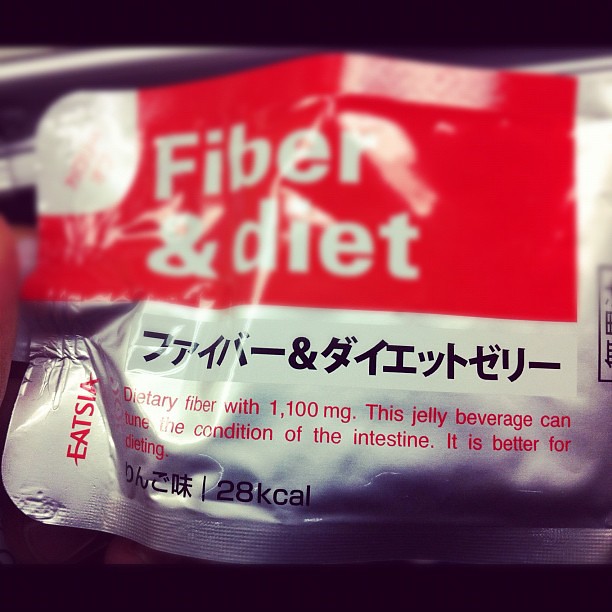A photograph captures a packaged food product in a sleek, gray foil pouch. The top-right corner features a prominent red bar with the words "Fiber and Diet" in bold white text. Below, on the silver section of the packaging, "Dietary Fiber" is highlighted in red text, emphasizing its content of 1,100 milligrams. This jelly beverage is formulated to aid in intestinal health and is marketed as beneficial for dieting, containing only 28 kcal per serving. A semi-circular area within the red bar is designed as a grip for easy opening, facilitating convenient use.